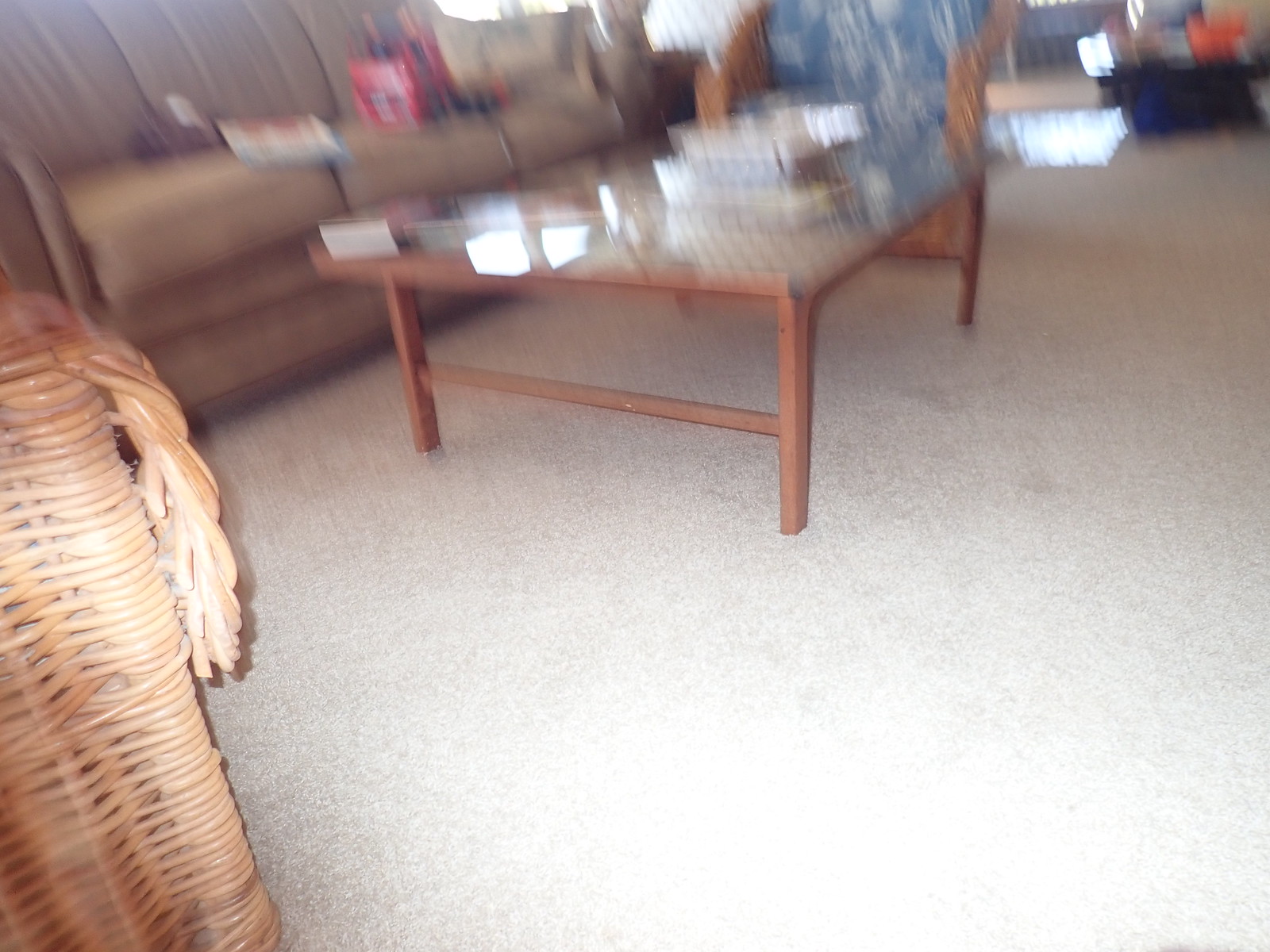The photograph captures a blurry interior scene, likely in the living room of a home. The image suggests that the camera was moved during the shot, resulting in an unclear depiction. The room features a light-colored carpet and is centered around a coffee table with wooden legs and a glass top. While the blur obscures the specific items on the table, they appear to be various objects, potentially books. Behind the table stands a tan-colored couch, cluttered with indistinguishable items, including at least one cushion or pillow and additional objects in red and black hues. To the left, partly visible, is a piece of wicker furniture that appears to be a chair. Adjacent to the coffee table and couch is another wicker chair adorned with blue and white cushions. In the background, darker-colored furniture pieces are faintly discernible, adding depth to the room's setting. Despite the blur, the composition hints at a cozy, lived-in space.